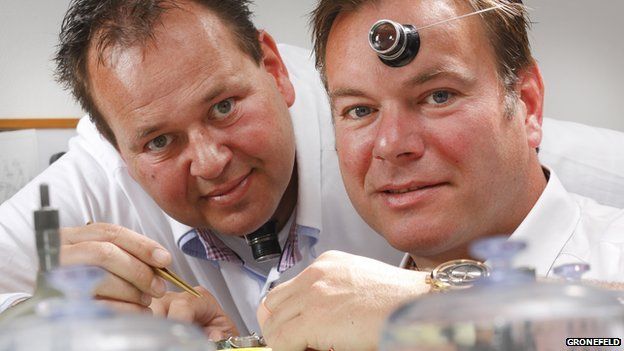The image depicts two middle-aged white men, likely scientists or jewelers, dressed in white lab coats. They are standing in a lab-like environment and looking directly at the camera. Both men are using different optical devices for close inspection. The man on the left, who has a slightly unsettling smile, has a stethoscope or microscope around his neck and holds a pointy gold instrument. He wears a white collared shirt. The man on the right smiles more pleasantly and has a magnifying lens on his forehead. He sports a fancy gold watch, and his hand rests on the table in front of them, where there is some sort of blurred equipment or container, possibly holding precious stones. Both men appear to be engaged in a detailed inspection with various instruments.